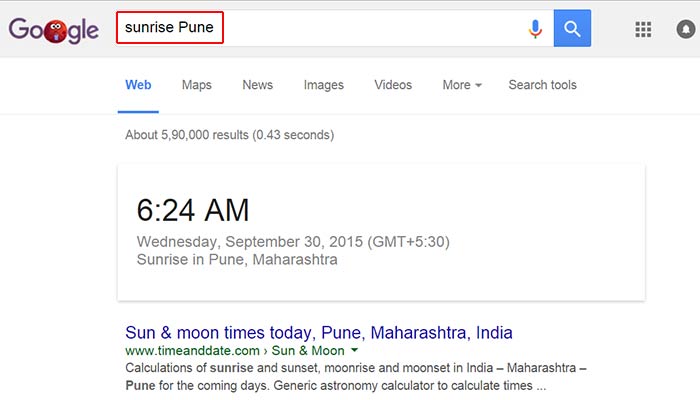Here is a detailed and cleaned-up caption for the image described:

"A screenshot of a Google Search page is shown, featuring a gray header bar at the top with the Google logo on the upper left. The logo has been customized to display 'Google' in purple, with the second 'O' modified to include a red icon with eyes. In the central white search bar, the search term 'Sunrise Pune' is highlighted by a red rectangular block. To the right of the search bar, there is a microphone icon and a blue search button. Additionally, to the far right, there are icons for grid pattern navigation and an alarm notification.

Below the header, the interface shifts to a white background area with navigation options including 'Web,' 'Maps,' 'News,' 'Images,' 'Videos,' and 'More,' accompanied by a dropdown menu and 'Search tools.' The 'Web' option is highlighted in blue, indicating the current selection. 

Further down, the search results indicate 'About 5,900,000 results in 0.43 seconds.' The primary result displayed is a time listing: '6:24 AM, Wednesday, September 30th, 2015, GMT +5:30, sunrise in Pune, Maharashtra.' Additional information from www.timeanddate.com includes details on 'Sun and moon times today, Pune, Maharashtra, India,' and provides calculations of sunrise, sunset, moonrise, and moonset times for Pune, Maharashtra, India, along with a generic astronomy calendar for future dates."